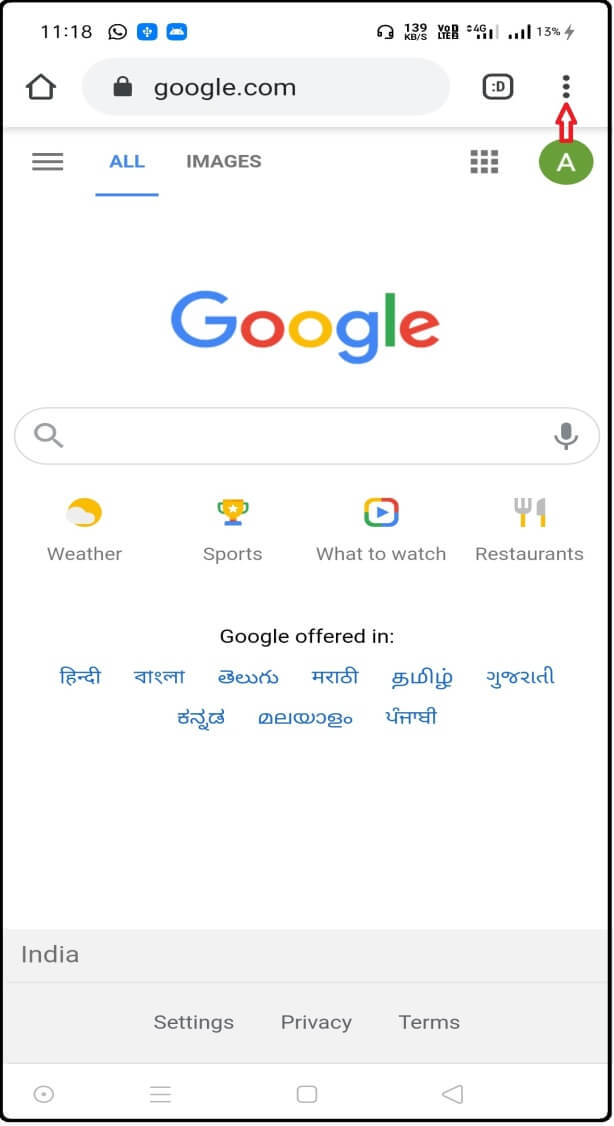The image is a screenshot taken from a smartphone, displaying the Google homepage. At the top, the time is shown as "11:18". There is an assortment of icons indicating connectivity and battery status: a signal strength indicator, a 4G icon, a battery symbol showing 30% charged with a charging symbol.

Below these, there's a search bar with three vertical dots, which when clicked, opens up settings for editing and format changes. The search bar is currently empty.

To the right of the search bar is a green circle with an upward-facing arrow, indicating an upward trend or perhaps an upload feature. This display is taken from the Google website.

On this Google homepage, there are several images representing different categories: 
1. A weather image showing a cloud and sky.
2. A sports icon represented by a trophy.
3. A 'What to Watch' section, indicated by a play button with a rainbow.
4. A restaurant section.

Additionally, the bottom of the page indicates that the user is in India; therefore, the page is available in multiple Hindu languages. 

Towards the bottom left corner, there is a search icon in a grey box. Centered just below this, the options 'Settings,' 'Privacy,' and 'Terms' are listed.

In the bottom left corner, there is a circle with a dot in the middle, next to three lines (likely a menu button), a square (perhaps representing recent apps), and a back button.